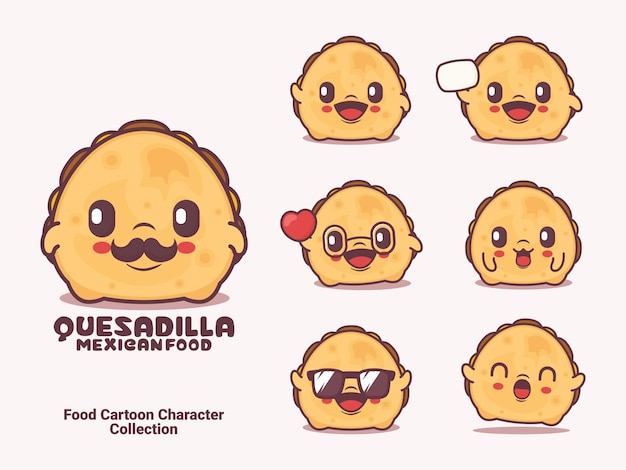The image showcases an advertisement for a Mexican food business, set against a light pink background. Dominating the left side is a larger cartoon quesadilla character with a rounded top and flat bottom, featuring large oval-shaped brown eyes, a black mustache, red dots on its cheeks, and a cheerful smile. Above this character, the text reads, "quesadilla Mexican food" in large brown letters, followed by "food cartoon character collection" below it. To the right, there are two vertical rows of three smaller quesadilla characters, each with distinct features and expressions. The top-left character in these rows wears black sunglasses and smiles widely, while the one to its right holds a white object. The middle-left character dons glasses and displays a red heart, and its right-side counterpart has its tongue sticking out like a playful dog. The bottom-left character is singing, and the bottom-right one sports sunglasses. All characters convey a joyful and lively demeanor.